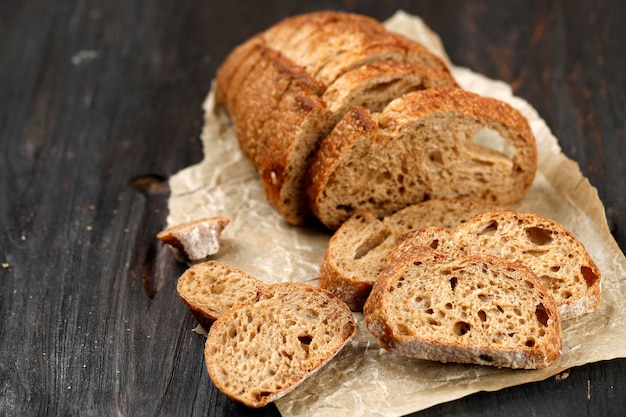A rustic, homemade-style loaf of bread, light brown in color with a crispy, hole-ridden texture, sits sliced on a crinkled and ripped piece of parchment paper. The parchment paper, resembling brown wax paper, contrasts with the dark, wood grain table beneath it. The loaf, wide and oval-shaped, has been partially sliced, with six pieces arranged neatly, and smaller end slices scattered haphazardly, leaving the rest of the loaf intact. The setting includes visible crumbs and signs of wear on the table, suggesting a dynamic and natural presentation of the bread. The clear, dynamic photo captures the fine details of the bread's texture and the rustic ambiance of the scene.